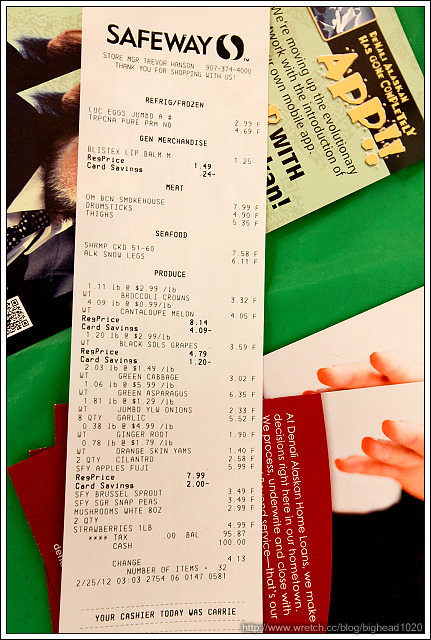The photograph captures a Safeway receipt positioned atop several flyers. The top flyer prominently features a message about Denali, Alaska, declaring, "Denali Alaskan has gone completely app," accompanied by an image of a chimpanzee in a business suit, symbolizing an evolutionary leap with the introduction of their new mobile app. The receipt obscures part of this flyer. The lower flyer promotes Denali Alaskan home loans, stating, "At Denali Alaskan home loans, we make decisions right here in our hometown. We process, underwrite, and close with," but the rest of the text is obscured.

The Safeway receipt, totaling $95.87, shows a detailed breakdown of purchases. It includes multiple sections: Refrigerated and Frozen, General Merchandise, Meat, Seafood, and Produce. The majority of the receipt is dedicated to produce, making up approximately 60% of the items listed. Additionally, there are two items under Seafood, three items under Meat, one item under General Merchandise, and two items under Refrigerated and Frozen. The transaction was completed with $100 in cash, resulting in $4.13 in change being returned to the customer.